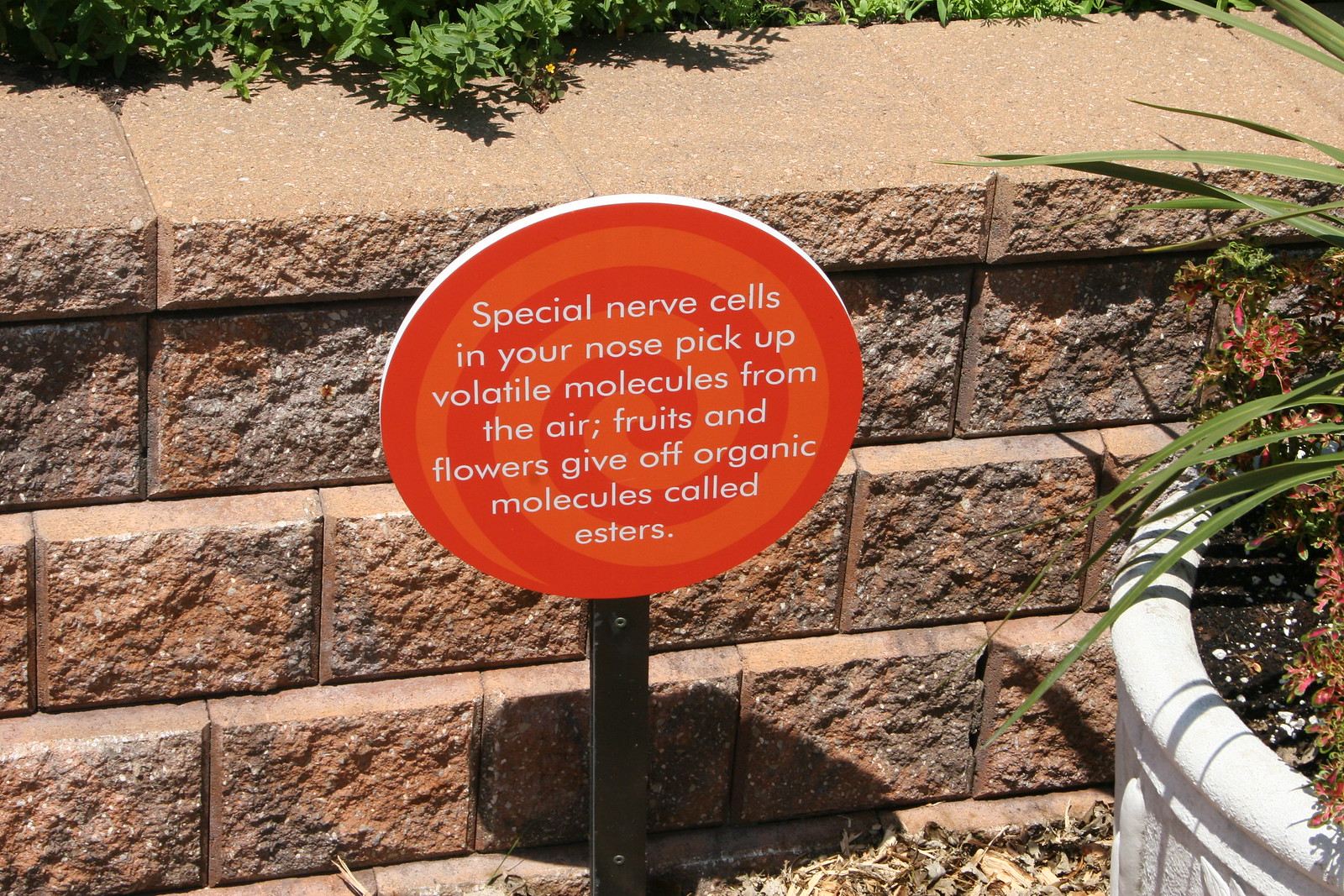The image depicts a vibrant outdoor scene, with the central focus on an informational sign situated in a garden or park setting. The sign, which prominently features a circular, lollipop-like swirl design in shades of red and orange, is mounted on a metal stand. It captures attention with its playful aesthetic, resembling a swirl candy, and is adorned with white text that reads, "Special nerve cells in your nose pick up volatile molecules from the air. Fruits and flowers give off organic molecules called esters."

Surrounding the sign is a well-maintained garden bed framed by brown stone or brick blocks, adding to the natural beauty of the setting. To the right of the sign stands a large, circular planter filled with various flowers and shrubs, enhancing the lush greenery of the area. In the background, a low brick or cement block wall can be seen, with more foliage visible beyond it, lending a serene and layered backdrop to the scene. This picturesque setup suggests a modern-day park aimed at educating visitors about the sensory processes related to plants and flowers in an engaging manner.